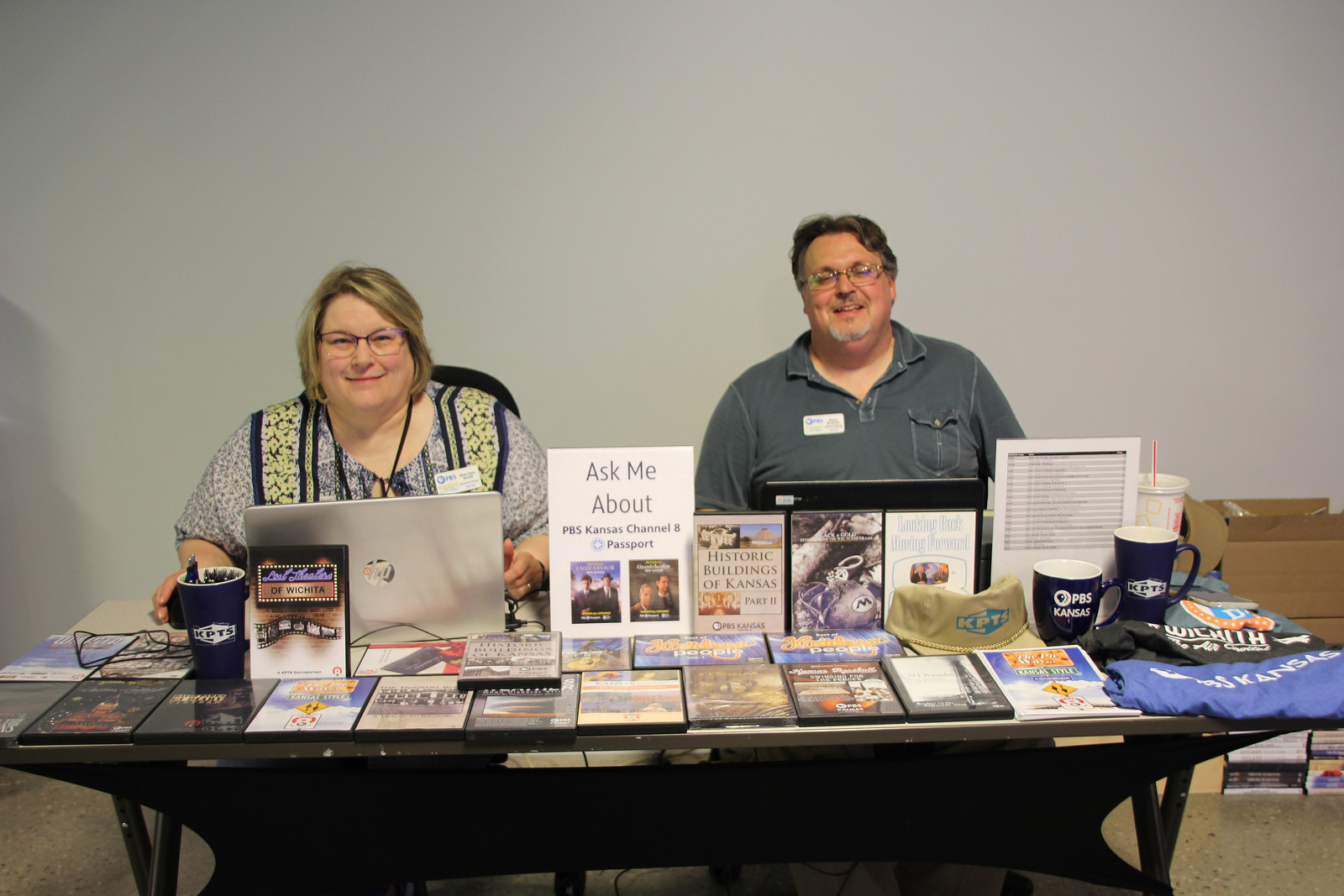In this image, a man and a woman are seated at a fold-up table set up for an event, showcasing a display for the PBS Kansas Channel Passport. The pair are both somewhat heavyset and wear name tags. The woman, positioned on the right, has chin-length blonde hair and sports a blue and white blouse under a yellow and blue patterned vest. She is focused on her laptop. The man, with brown hair, glasses, a white beard, and a gray shirt with a front pocket, appears to be more relaxed and laughing. 

On the table, there is a prominent sign that reads "Ask me about the PBS Kansas Channel Passport." In front of the sign, a collection of DVDs starts from the left side, alongside books and a cup holding pens. A DVD or sign notably mentions Wichita. On the right side of the table, various promotional items are displayed, including two black coffee mugs with white lettering, a hat, and additional tchotchkes.

The background behind the pair is a plain, light gray, drawing attention to their colorful display of merchandise and promotional materials.